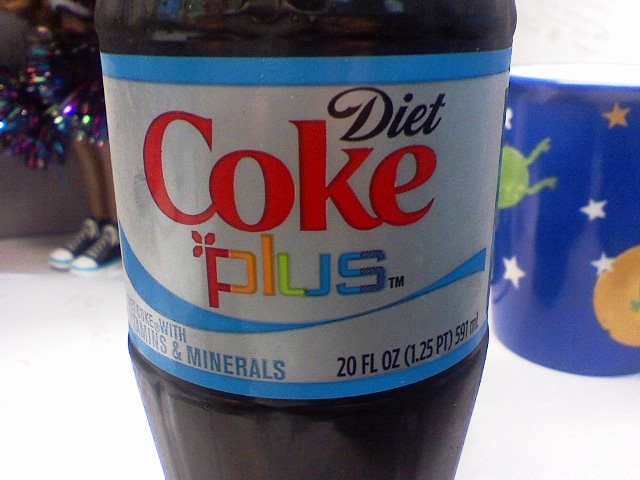This photograph depicts a 20-ounce bottle of Diet Coke Plus prominently displayed against a white floor background. The bottle, made of reflective plastic, contains dark brown soda visible through its clear exterior. The label of the bottle features a predominantly silver-gray background with medium blue bands at the top and bottom. The word "Diet" is inscribed in black cursive text, followed by "Coke" in vibrant red, and "Plus" in a gradient of red, orange, yellow, light green, medium blue, and dark blue. Accompanying the word "Plus" is a small black "TM" and a medium blue swoosh below it, leading to some text partially reading "Coke with Timmins Ampersand Minerals." Additionally, at the bottom right of the label, the volume is noted as "20 FL OZ 1.25 PT 591 ML."

Set against this central figure, on the right side, there is a cobalt blue mug featuring a design with stars—both gold and white—and spherical, possibly planetary, shapes, one orange and another green. This mug adds a whimsical, cosmic touch to the scene. In the top left corner of the image, a pair of human legs are visible, adorned with black Chuck Taylor shoes that have white tips and laces. These legs appear to be holding multi-colored iridescent pom-poms, adding a splash of vibrant color and a playful element to the composition.